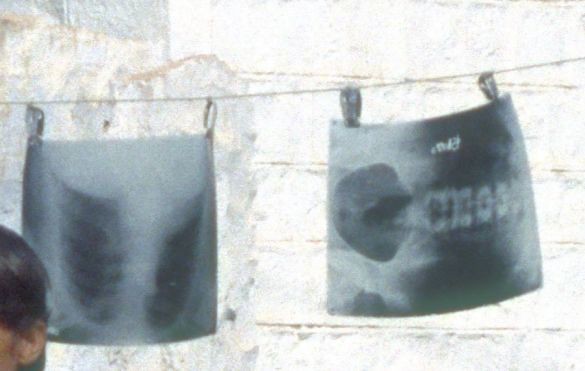In this color photograph of exceedingly poor quality, a dim and fuzzy background, primarily gray with hints of brown and black, partially obscures a scene. A thin, faded line or string stretches horizontally across the composition, from the upper right corner to the middle left, with two x-rays hanging from it. The left x-ray displays a torso and ribcage, while the right features a pelvis and lower spine. In the lower left-hand corner, a dark-haired, dark-skinned individual can be seen, identifiable only by their left ear and part of their head, which might be partially obscured by a green mask. The setting appears to be outdoors, with the back wall potentially lit by natural light.